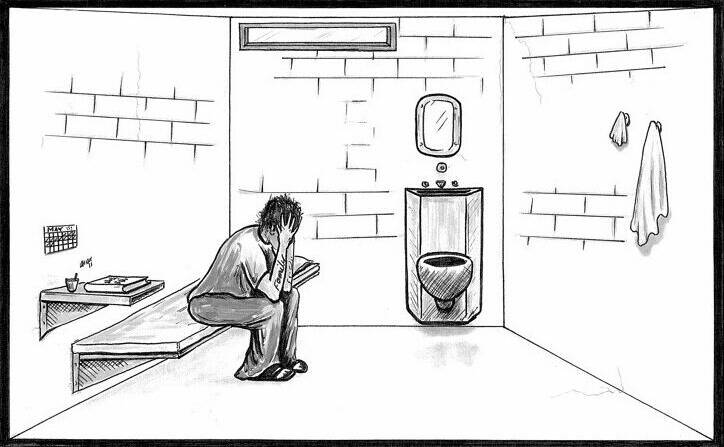The black and white image is an artistic drawing of a small jail cell. The horizontally rectangular frame includes a black border, while the interior remains stark and white, resembling a blank screen. Within this constrained space, a young man sits on a simple bench-like bed, his head cradled in his hands, conveying a profound sense of despair. 

The cell's walls, constructed from concrete cinder blocks, define three sides of the image. The left wall features a floating shelf above the bed, holding a solitary book and a glass. Directly above the man is a slim, horizontally rectangular window, allowing only a sliver of light to penetrate the gloom. Attached to the back wall is a combination sink and toilet unit, with a small mirror positioned above it. The right wall is adorned with two towels hanging neatly. The floor of the cell remains notably unmarked, reinforcing the oppressive emptiness that characterizes the scene. Items such as a calendar further emphasize the passage of time in this desolate environment.